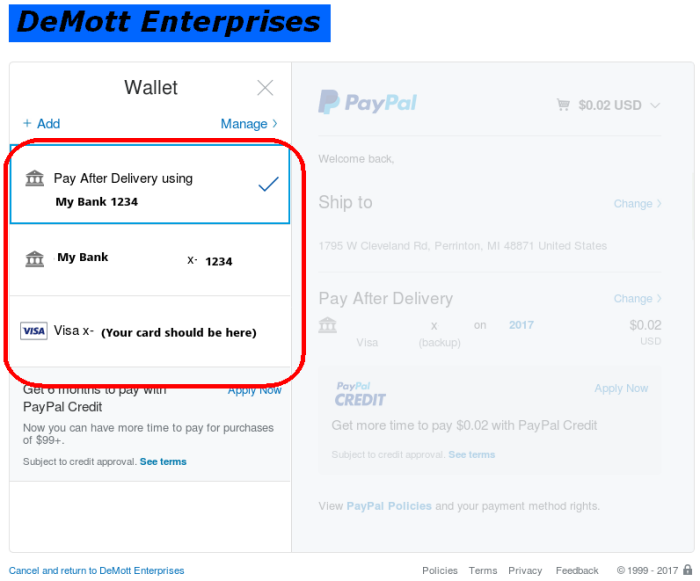The image depicts the interface of a financial transaction screen, split into two sections. 

In the top left corner, a blue rectangle features the text "Demat Enterprises" in black. Below this, the PayPal section begins, divided into two columns. On the left, at the top, is the word "Wallet" followed by options to "Add" and "Manage" in blue text. Within the "Manage" section, there is a gray X icon. Below this, it displays "Pay After Delivery using my bank 1234," marked with a blue check mark. This selection is highlighted with a red square. Additional information below includes "My bank 1234" and "Visa X," with a note indicating where the card details would be shown.

Further down, a prompt reads "Get six months to pay with PayPal Credit. Apply now," allowing users more time for purchases over $99. This area has a gray background.

In the right-hand section, the top features the PayPal logo, which transitions from blue to light blue. Below this, the balance reads "0.02 USD" followed by text welcoming the user back, along with an option to change their shipping address. The section includes the current address and mentions the "Pay After Delivery" option again. At the bottom, "PayPal Credit" is emphasized with the note, "Get more time to pay 0.02 with PayPal Credit."

Further below, it advises the user to "View PayPal policies and your payment method rights." In the bottom right corner, four categories are listed: "Policies," "Terms," "Privacy," and "Feedback." At the very bottom right, it reads "1999 to 2017" next to a lock icon, indicating the range of years and security assurance.